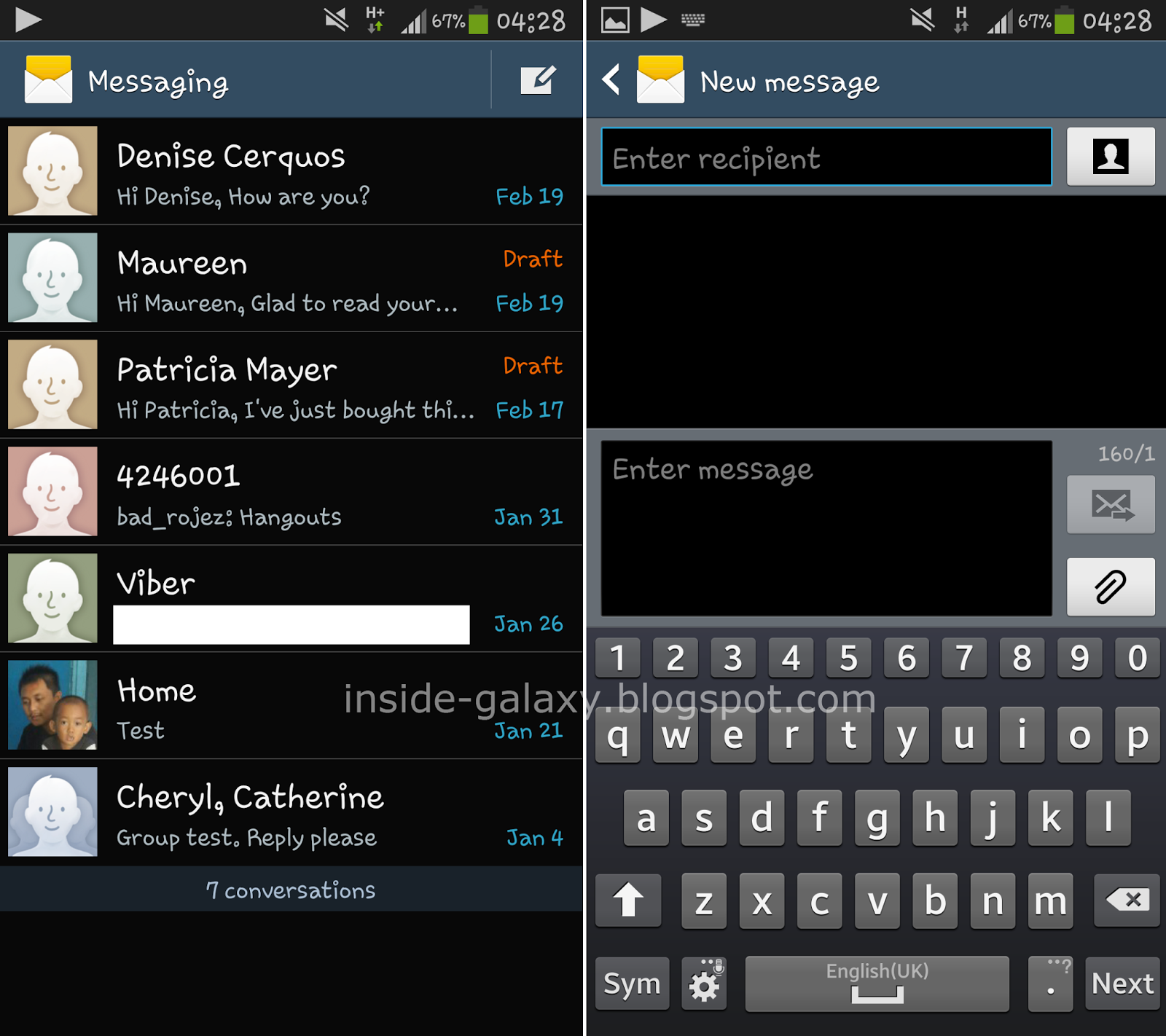The image consists of two side-by-side screenshots from a smartphone. 

The left screenshot features a black background. At the top-left corner, there is a play button icon. Adjacent to it, the battery indicator displays 67%, and the time is shown as 4:28. Below this, a gray bar labeled "Messaging" appears, with an envelope icon on the left and an icon resembling a piece of paper with a pencil on the right. The main section below this bar shows a list of contacts, each displayed as a square with a profile picture. Most of these profile pictures are default blank avatars, except for the second contact from the bottom, which shows an image of two children. The highlighted contact is named "Viber," and appears to be in the process of composing a message, indicated by a typing bar under the name.

The right screenshot displays a popup window titled "New Message." It prompts the user to "Enter recipient" and "Enter message," with respective input boxes for each. The smartphone's keyboard is activated at the bottom of the screen, suggesting that the user is about to type a message.